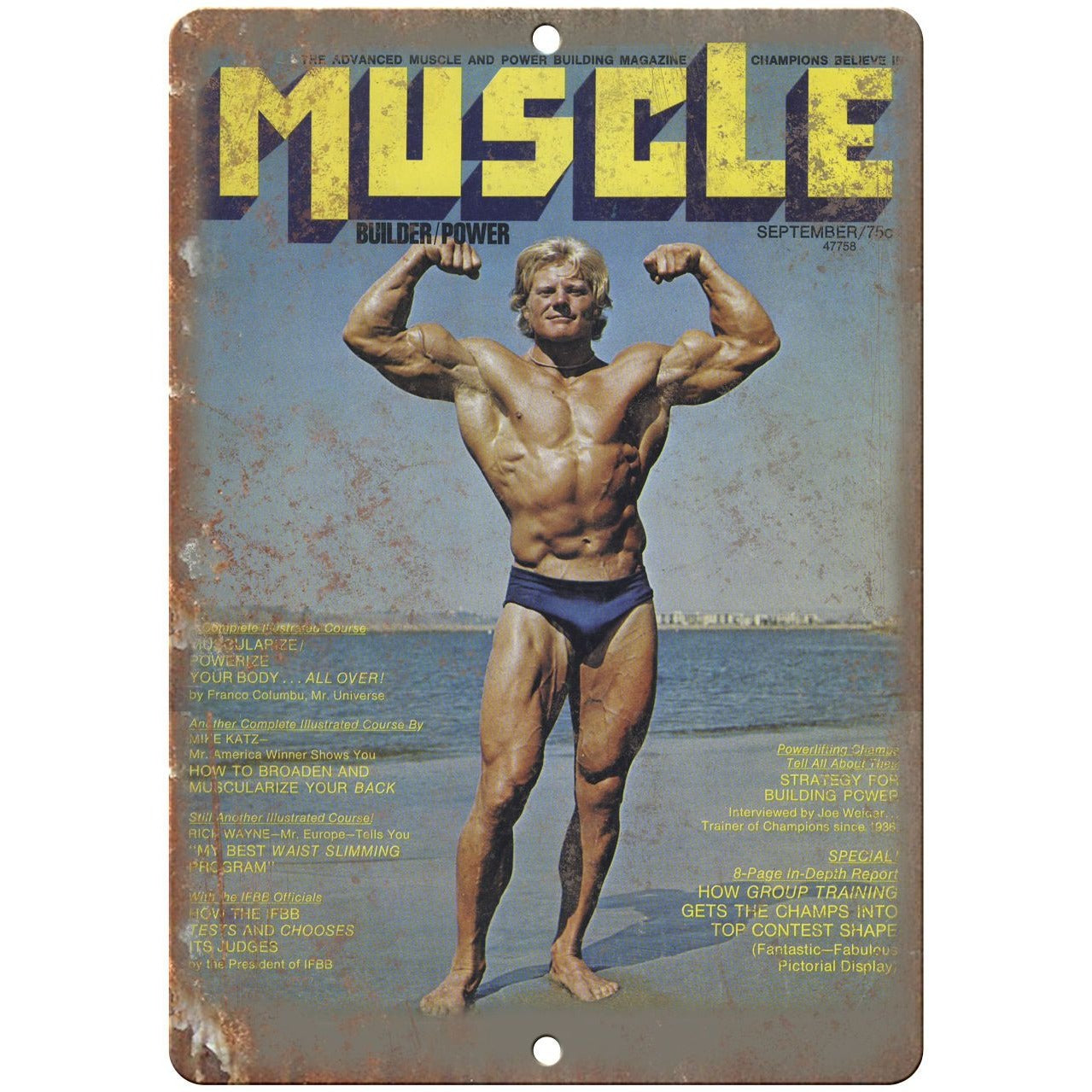This image features a retro-look metal sign resembling the cover of the "Advanced Muscle and Power Building" magazine, titled "Champions Believe in Muscle Builder/Power." This edition, dated September '75 (issue 47758), prominently displays bodybuilding icon David Draper. Draper stands confidently in a blue bikini bottom at a beach shoreline, striking a classic bodybuilder pose with both arms flexed and his bushy blonde hair blown by the wind. The backdrop includes a serene blue sky and dark blue water, with a distant cityscape appearing faintly on the right. The wet sand beneath adds to the nostalgic 70s ambiance, enhanced by the image's faded sunny hues.

The cover is laden with bright yellow text, showcasing various article titles on the left, such as "Complete Illustrated Course: Muscularize, Powerize Your Body All Over" by Franco Colombo, Mr. Universe, and a guide by Mike Katz, Mr. America Winner, on how to broaden and muscularize your back. Additional features include Rick Wayne, Mr. Europe, offering his best waist-slimming program, and insights about how the IFBB tests and chooses its judges by the IFBB President. Below Draper’s feet is a notable white dot and text mentioning a special 8-page in-depth report on group training strategies by Joe Weider, renowned trainer of champions.

The metal sign has two small nail holes at the top and bottom, suggesting it might be mounted. Rust along the edges adds to its retro charm, making this piece both a striking visual and a rich historical artifact of vintage muscle magazines.